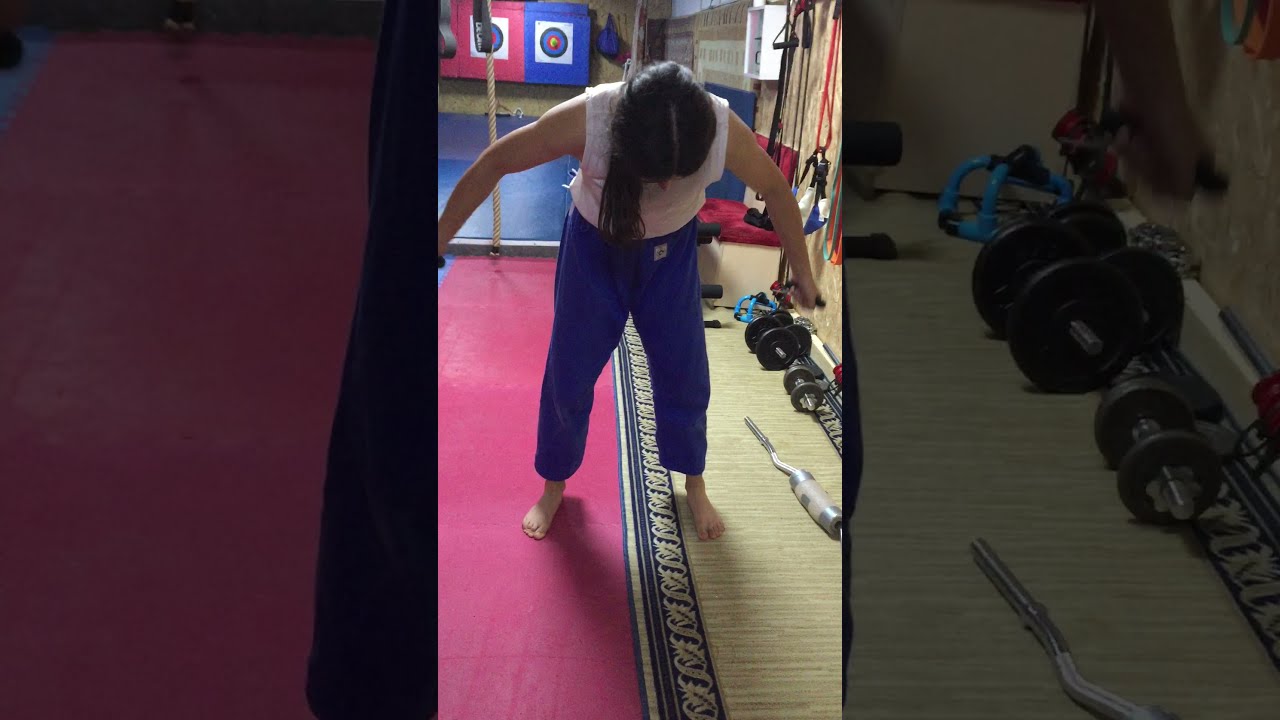In this image, a young woman, possibly in her late teens or early twenties, is captured in a gym environment. She has long, dark black hair that cascades down as she leans forward slightly, her head bowed. Dressed in a white sleeveless tank top and blue sweatpants, she is barefoot, standing on a floor that features patches of red and blue, with a carpet-like section showing a fancy leaf pattern. The woman's arms are extended wide, gripping resistance bands which she is pulling towards the center of her torso in a flexing motion. To her right, the gym wall is adorned with various pieces of equipment including jump ropes, dumbbells, stretchy bands, and what appear to be bullseye targets in the background. The gym setting around her is cluttered with weights and ropes, enhancing the sense of a busy, well-used workout space.